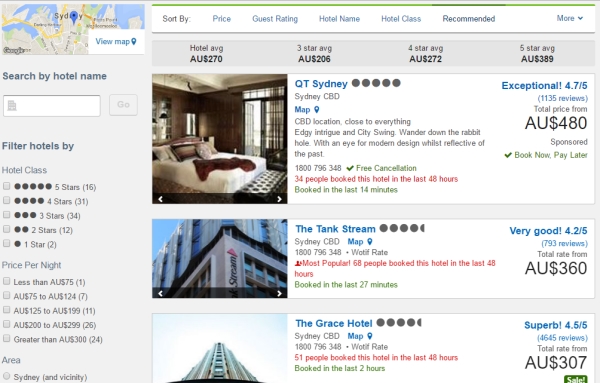The image depicts a detailed search for hotels in Sydney, Australia. In the upper left-hand corner, there is a map highlighting Sydney with a prominent blue circle, indicating the search's focal point. Filters are displayed prominently on the left side of the screen, allowing users to narrow their results by hotel name, star rating, price per night, and area.

The star rating filter includes options for one to five stars, with the number of available hotels listed in parentheses next to each rating. The price filter is segmented into ranges that start at $75 AUD, progressing to $75-$124 AUD, $125-$199 AUD, and so on. The area filter currently only shows "Sydney and vicinity."

Three hotel listings are visible in the search results:

1. **QT Sydney**: This hotel boasts a five-star rating with an exceptional score of 4.7 out of 5 based on 1,135 reviews. The nightly rate is $480 AUD. The listing is described with phrases like "edgy," "intrigue," and "city swing," inviting guests to "wander down the rabbit hole with an eye for modern delight."

2. **Tank Stream Hotel**: With a 4.5-star rating and a "very good" score of 4.2 out of 5 from 793 reviews, this hotel is priced at $360 AUD per night.

3. **Grace Hotel Sydney**: Also with a 4.5-star rating but labeled "superb," this hotel has an impressive review score of 4.5 out of 5 from 4,645 reviewers. It is the most affordable option among the three, costing $307 AUD per night.

Overall, the webpage offers a comprehensive overview of high-rated hotel options in Sydney, complete with specific details to aid in the decision-making process.